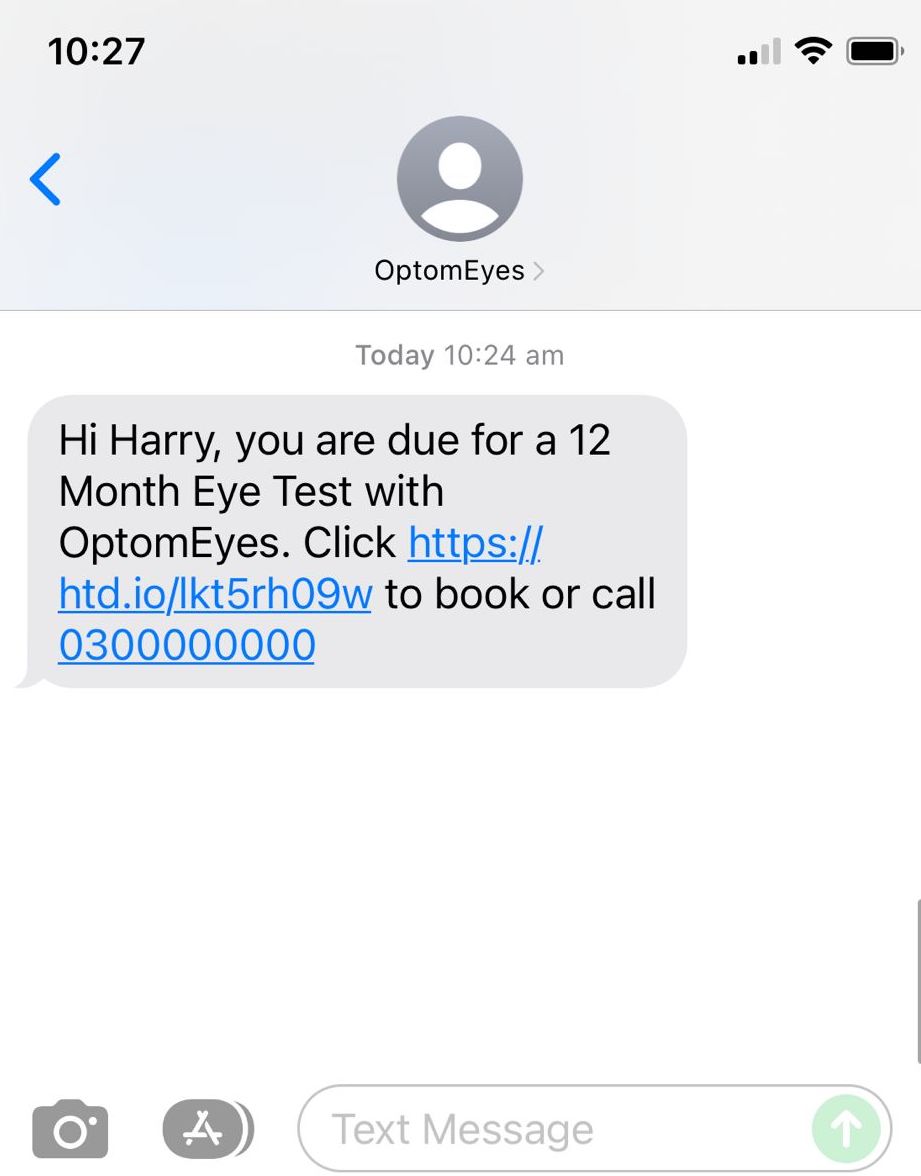This image, captured from someone's phone screen, displays the interface of a messaging application. At the top, there is a gray status bar. In the upper left-hand corner, the time is displayed as 10:27 in black text. The central portion of the status bar is empty, while the right side features several icons including signal bars, a Wi-Fi symbol, and a fully charged battery icon depicted in black.

Below the status bar, there is a blue back arrow pointing left. Centrally aligned is a silhouette of a human figure next to the text "OptumEyes," accompanied by a faint gray forward arrow to the right.

In the main white section of the screen, the message timestamp reads "Today, 10:24 AM." Below this timestamp, a gray speech bubble contains the following message:

"Hi, Harry. You are due for a 12-month eye test with OptumEyes. Click https://http.io/IKT5RHOW to book or call," followed by a phone number.

Each clickable element, the URL link, and the phone number is highlighted, indicating they are interactive.